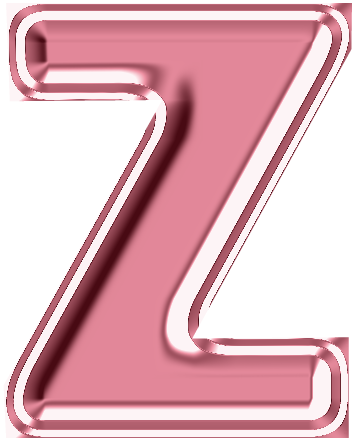The image is a digital artwork featuring a capital letter "Z" in the center of a white background. The "Z" appears to have a 3D effect with a slightly recessed look, enhanced by a shadow on the left side, which adds to the depth perception. The interior of the "Z" is filled with a dark pink, almost red color, giving it a vibrant appearance. This central dark pink section is bordered by a thin white outline, which is itself outlined by a darker pink trim. The right side corners of the "Z" are highlighted with extra dark pink, and they appear to be slightly rounded with a squared-off section, adding complexity to its shape. The design also features a subtle shine on the lower sections of the top and bottom parts of the "Z," contributing to its glossy, metallic look.